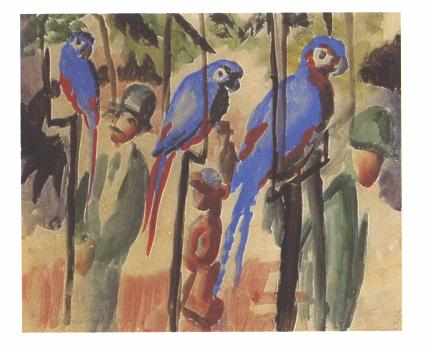The painting, likely done in acrylic, depicts a scene featuring three vibrantly colored blue parrots with red tails perched on black sticks being held by human figures. The parrots vary slightly in size and color: the one on the right has a predominantly red chest with red feathers and a white area around the eyes tinged with red. The central parrot shows a mix of black and red in the same areas, while the one on the left is distinctively blue with a red body and a clear white face. The birds are positioned with one on the left facing left but with its head turned to the right and the other two facing right. The human figures, likely army soldiers, are dressed in green outfits and metallic-colored hats, some looking at the parrots while others face away. The background is a tan color with green and black specks mimicking grass and rocks, lending the image an earthy, muted tone that contrasts with the vivid colors of the parrots. There is no visible artist's signature in the painting.